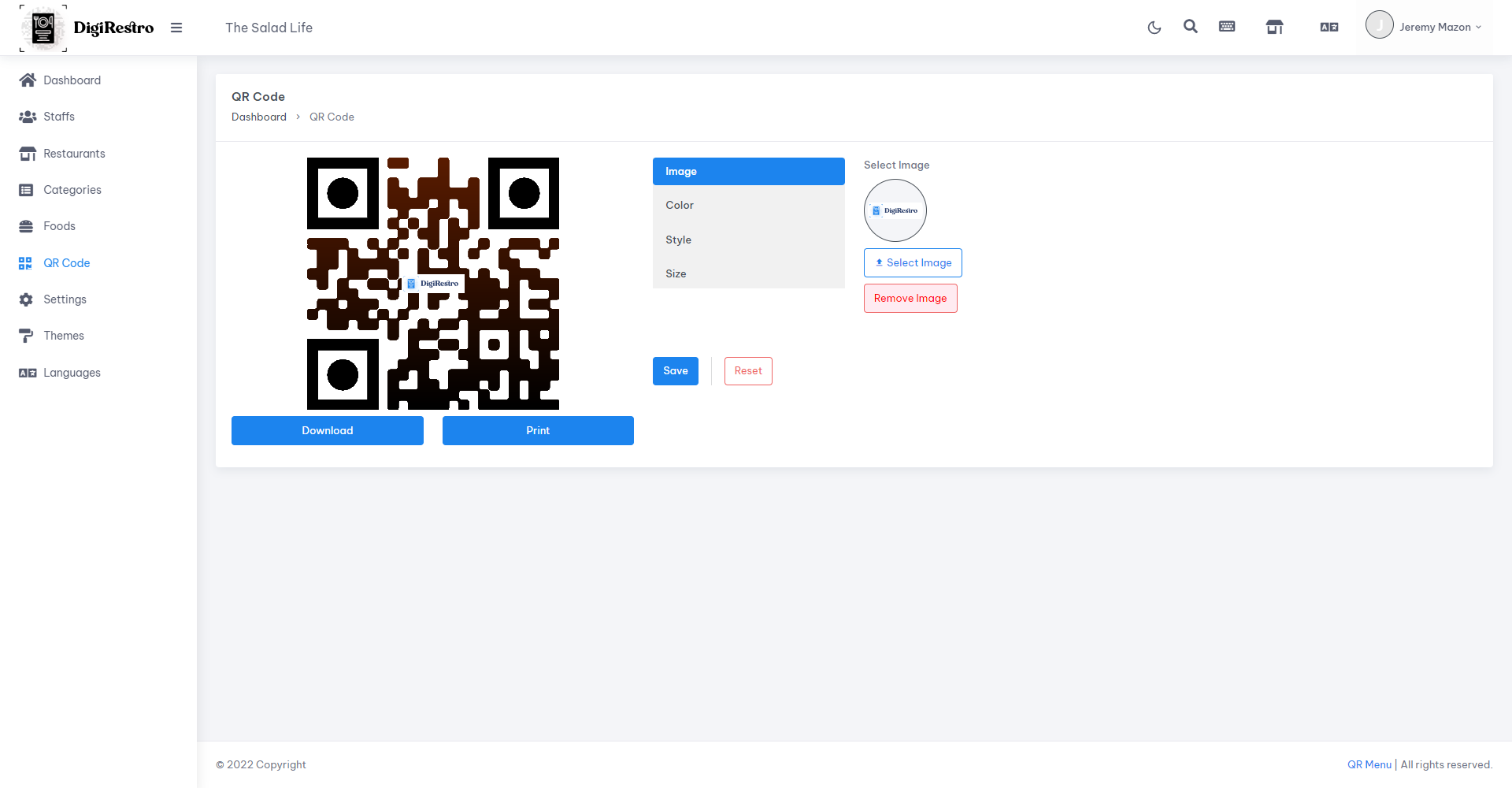In this screenshot of the Digi Restro interface, the top left corner prominently displays "Digi Restro" in black text. To the right, "The Salad Life" is written in light gray, both standing out against the white background. At the top of the screen, there are various icons including a half moon, magnifying glass, home icon, keyboard icon, and two small blocks with dots, whose function is unclear. A circular profile picture with a 'J' in the center is also visible, indicating the profile of Jeremy Mozos, though his full name is hard to read.

Below these elements is a section containing a QR code labeled "dashboard QR code." This QR code can be downloaded or printed and is currently selected under the "image" option. There are additional options for "color" and style and size adjustments. Users can choose to save or reset the configurations.

On the left side of the screen, there is a navigation panel in gray, featuring icons and labels. These include a home icon labeled "dashboard," a people icon labeled "staff," a building icon labeled "restaurants," a list icon labeled "categories," and a square blob icon labeled "foods." The "QR code" option is highlighted in blue. Further down, there are icons for "settings" represented by a gear, "themes" represented by a paintbrush, and "languages" marked with an alphabet-like icon.